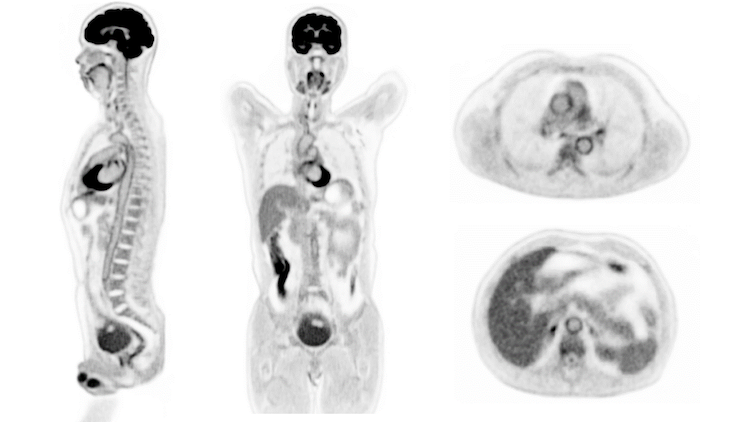The image features four distinct MRI scans of the human torso, presented in two sets, each showcasing different perspectives and sections. 

The first set, on the left, includes two sagittal MRI slices:

1. The upper-left image is a sagittal slice taken from the left side of the torso, cutting through the midline. This detailed scan vividly displays the brain, spinal cord, heart, and bladder, clearly delineating major anatomical structures from this side angle.
   
2. The lower-left image is a coronal slice, offering a frontal view of the torso, yet again cutting through the midline. This view highlights the brain, nasal passages, heart, lungs, liver, and possibly the bladder, providing a comprehensive look at the torso's internal organs from the front.

The second set, on the right, comprises two axial MRI slices:

3. The upper-right image shows an axial section taken through the abdomen, revealing structures around the spinal cord. This slice captures various abdominal organs, muscle, and fat layers, although specific organs are not distinctly identifiable to the untrained eye.
   
4. The lower-right image, another axial slice, offers a similar view of the abdomen, showing the arrangement of the spinal cord, muscles, fat, and surrounding organs. Again, precise identification of these anatomical features might be challenging without advanced medical knowledge.

Overall, this set of MRI images provides an intricate and multidimensional view of the human torso, highlighting various anatomical structures from different orientations.